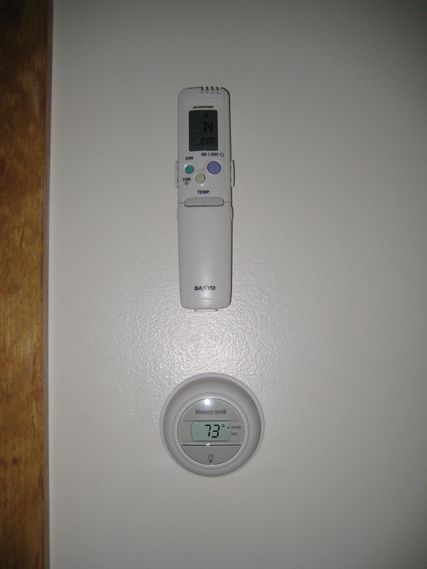In the image, a Sanyo remote control is prominently displayed on a white wall. The remote is elongated and rectangular, featuring several buttons arranged on its surface. Notably, it includes three or four round buttons toward the top and a small square display screen. Directly beneath the screen, there is a large rectangular button for adjusting settings, flanked by up and down arrows on either side.

Positioned below the Sanyo remote is a Honeywell thermostat, also mounted on the same white wall. The thermostat has a round, circular design and displays the current temperature reading of 73 degrees on its digital interface, accompanied by a small light bulb icon.

To the left of both the remote and the thermostat, a wooden panel adds a contrasting texture to the scene. The overall composition places these two functional devices—one for controlling temperature settings via the remote and the other for monitoring the room temperature—on a minimalist, white backdrop, emphasizing their utilitarian roles.